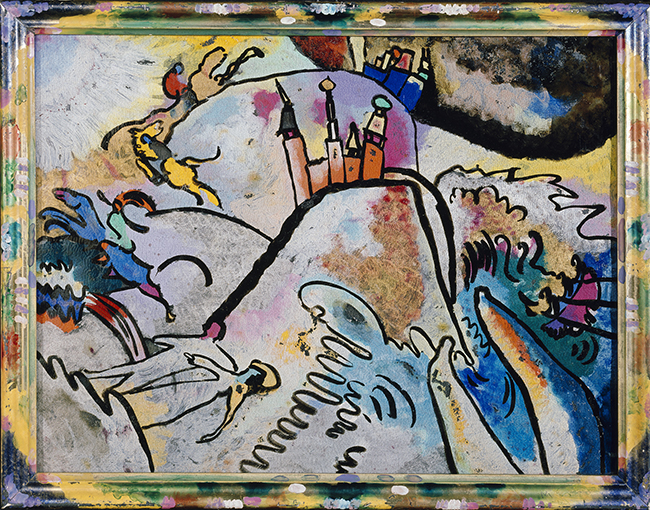This expressive abstract painting, potentially by Wassily Kandinsky, is a vivid canvas alive with multifaceted elements and a rich palette of colors including blue, green, yellow, red, and orange. Dominated by a large central form, reminiscent of an upside-down U akin to a mountain or castle, the scene is densely packed with various smaller motifs. Among these are discernible figures such as people and horses, which may evoke the image of the Four Horsemen of the Apocalypse. Buildings reminiscent of Russian architecture with onion dome tops dot the landscape, merging seamlessly with an assortment of abstract forms like waves, squiggly lines, and even a whale leaping from water. The painting’s tactile brush strokes contribute to its dynamic and chaotic energy, incorporating possible depictions of people dancing, a dog leaping, and a sea creature. A sense of contrast is hinted at by elements portraying clean versus dirty air, symbolized by factories emitting smoke. The painting's abstract nature and multicolored, expressive style make it challenging to derive a singular message, yet its complexity and vibrancy captivate the viewer.